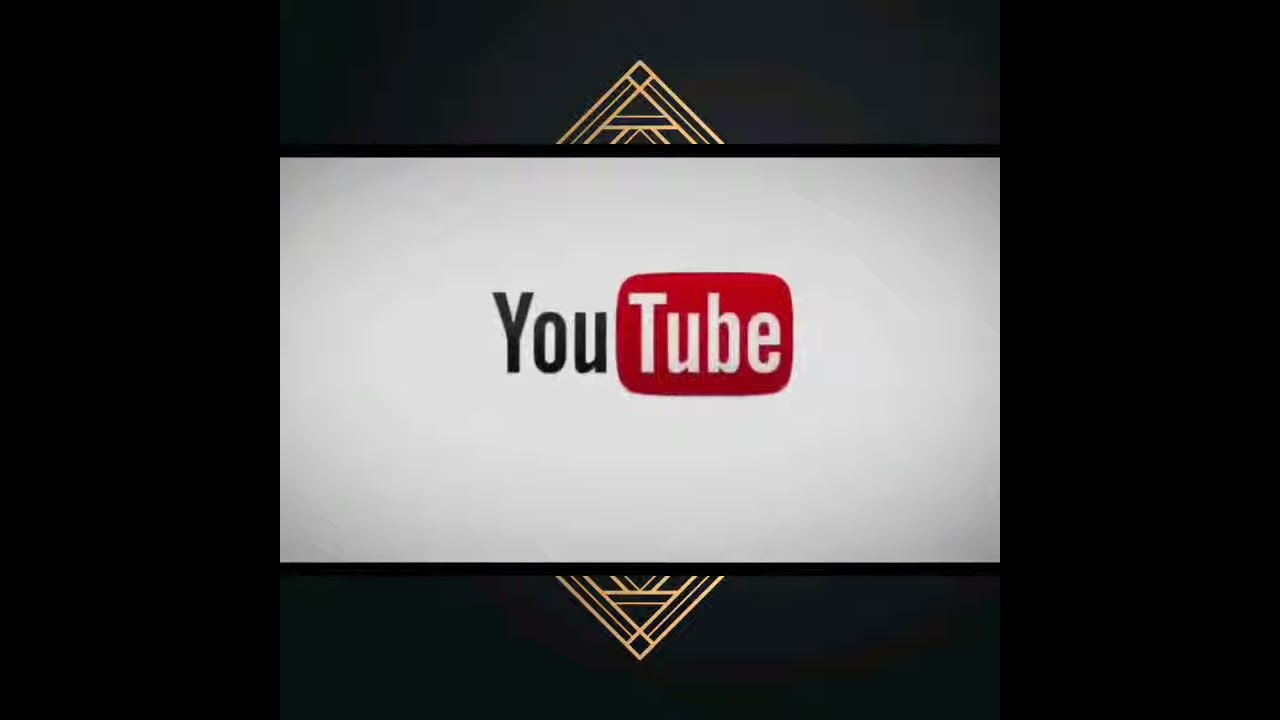The digital image features a stark black background, dominated by a central white rectangle. Within this white rectangle, the prominent YouTube logo is displayed. The logo consists of the word "YouTube," where the "You" is rendered in black letters, and "Tube" is depicted in white letters against a red backdrop. The YouTube logo text appears large and standard, accentuating its recognition factor. Above and below this central white rectangle are golden triangular shapes, with the top triangle pointing upwards and the bottom one pointing downwards. These triangles add a geometric pattern to the composition. Additionally, a thin black border outlines the white rectangle, further separating it from the dark background. The contrast is heightened by a subtle light source that gives the white part of the YouTube logo a slight glare, making it pop against the deep black and dark bluish-gray background.